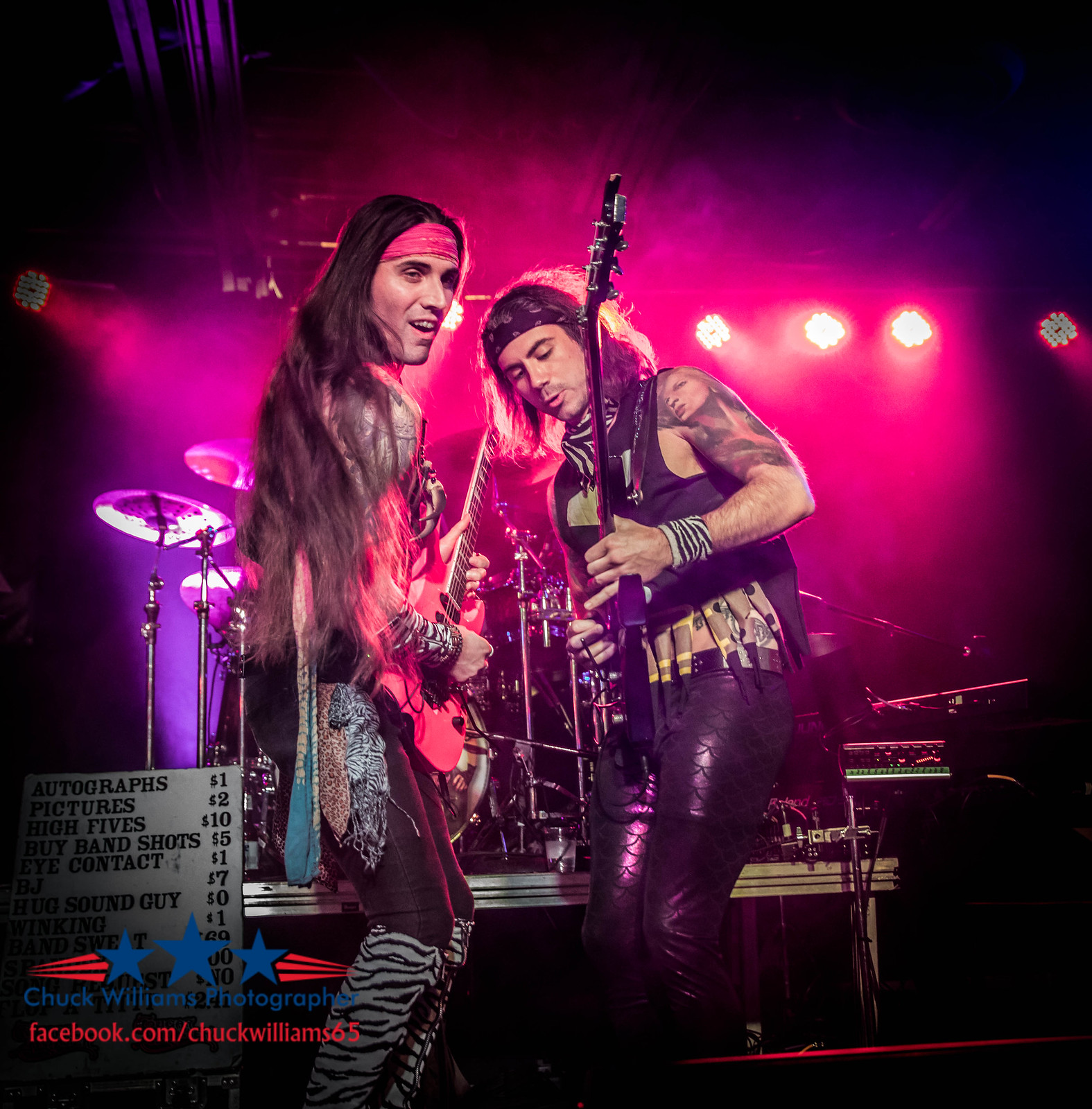In this vibrant image, two long-haired men are performing on a dimly lit stage, likely as part of a rock or metal band, framed by striking purple and pink spotlights. The man on the left, a white male with flowing dark brown hair, wears a red headband tied around his forehead. He's clad in a red shirt, black pants, and distinctive leopard-print boots, further accessorized with leopard-print handkerchiefs hanging from his pocket. He plays a pink electric guitar with focused intensity, his mouth open as he immerses himself in the music. His knees are slightly bent, adding a dynamic pose to his performance.

Next to him stands another white male with shoulder-length dark brown hair, accented by a black bandana. He showcases his arm tattoos, dressed in a black tank top and shiny black leather pants, all while playing a dark-colored electric guitar, likely a bass. His wrist is adorned with a wristband, potentially in an animal print pattern like zebra or leopard spots.

Behind them, the stage is equipped with a drum set and other musical gear, illuminated by an array of pink and purple lights that reflect off the performers, enhancing their glam rock image. The lower left-hand corner of the image features a partially visible whiteboard listing prices for autographs, pictures, high fives, band shots, and contact information. The photographer, Chuck Williams, is credited at the bottom left, with "Chuck Williams Photography" and his Facebook URL, adding a final touch to this vivid scene.